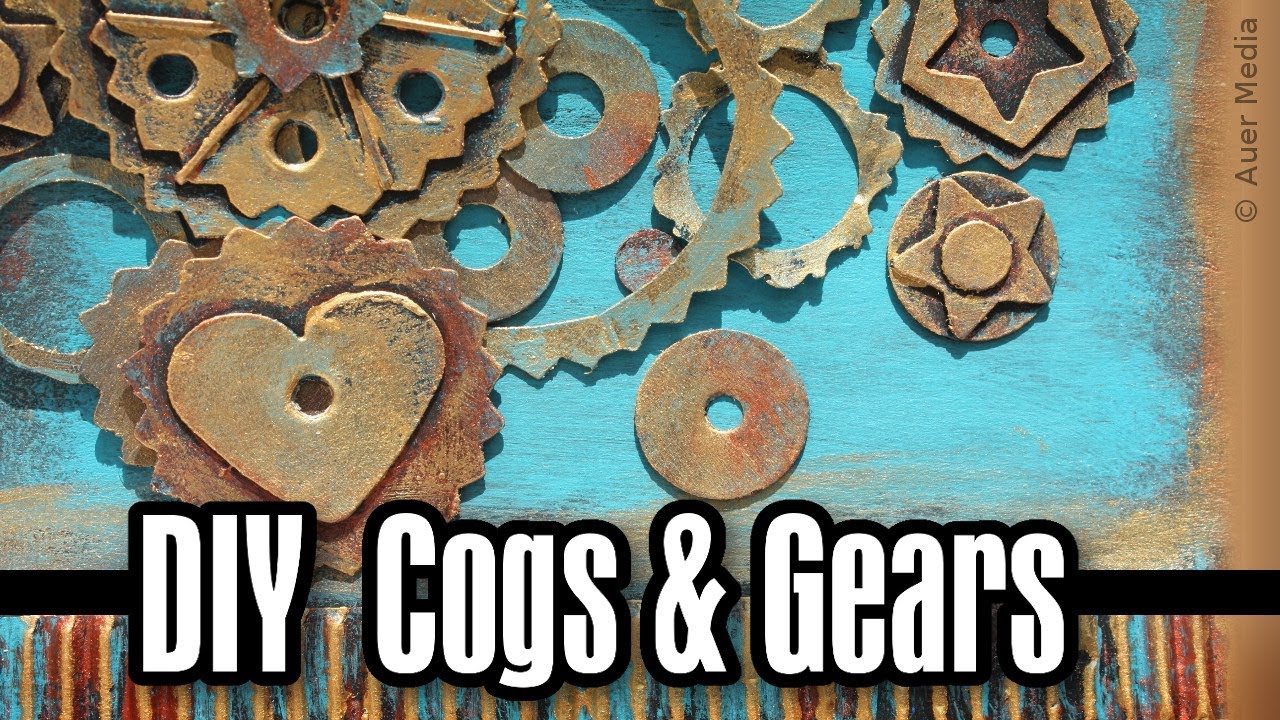The image presents an intricate advertisement for DIY cogs and gears against a textured light brown background, partially covered by a light turquoise spray paint. The brown background peeks through on the right side and bottom, creating visible borders of a few inches wide. The focal point features various gold and rusty-colored watch components, including circular bolts and intricate pieces, some uniquely shaped like stars and hearts.

In bold white letters, outlined in black, the text "DIY Cogs and Gears" spans the width of the image over the turquoise area. Below this, a series of alternating lines in turquoise, brown, red, and blue chalk traverse the overall width, adding a vibrant, creative touch. The right side of the image contains a vertical copyright watermark for "AUER Media," written sideways. The overall composition suggests a hands-on, creative approach to assembling detailed cog and gear designs from cardboard or similar materials, highlighted by the diverse and artistic paint applications used in their creation.